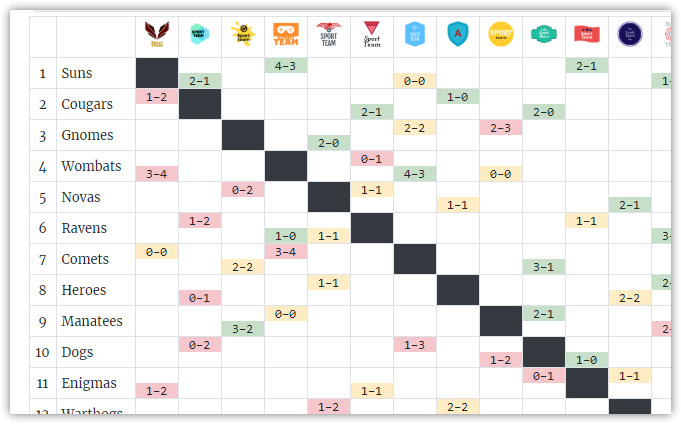This image presents a detailed diagram outlining the match outcomes for 12 teams. The layout features a white background with a thin gray line running horizontally across the top and another parallel line slightly below it. Vertically, a gray line approximately a quarter-inch from the left edge marks the start of a series of columns, with similar thin gray lines separating various sections of the table.

On the far left column, numbers from 1 to 12 are listed vertically. Adjacent to this, the next column contains the names of the 12 teams. At the top horizontal row, immediately to the right of an empty cell, the logos of these 12 teams are displayed from left to right.

The main body of the table, situated below the rows of team logos, consists of a grid of rectangles. Each cell in this grid represents the outcome of a match between the teams. The first column is labeled "1 Suns," and following its row to the fourth column shows an entry "4-3," indicating the Suns have played 4 matches and won 3. Similarly, continuing to the tenth column reveals an entry "2-1."

Color coding is used to indicate match outcomes: 
- Pink cells denote a losing record (e.g., 1-2).
- Blue cells indicate a winning record (e.g., 2-1).
- Tannish cells represent a tie (e.g., 1-1).

Diagonal black blocks traverse from top to bottom, marking the matches where the team name corresponds directly with its logo. This comprehensive layout provides a clear visual of how each team has performed against the others, including wins, losses, and ties.